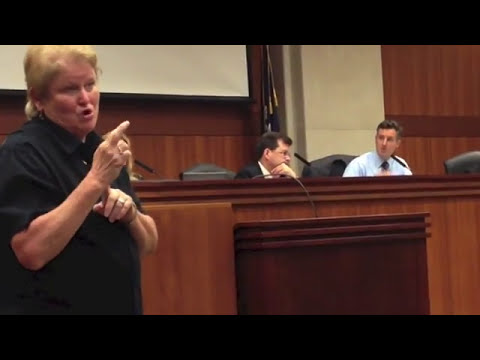This image, horizontally aligned with thick black borders at the top and bottom, is taken inside a courtroom. The scene features a brown-paneled wall with a white screen in the upper left-hand corner. In the foreground to the left, there is a middle-aged woman wearing a black shirt, gesturing with her right hand while her left arm rests on her chest. Behind her, the judge, seated centrally, is engaged in a conversation with a man in a blue button-down shirt and tie, who is positioned to his right. Both the judge and the man have microphones in front of them, and to the far right of the image stands a dark wooden podium with a long, curved microphone. A flag is also visible, adding to the official atmosphere of the courtroom.